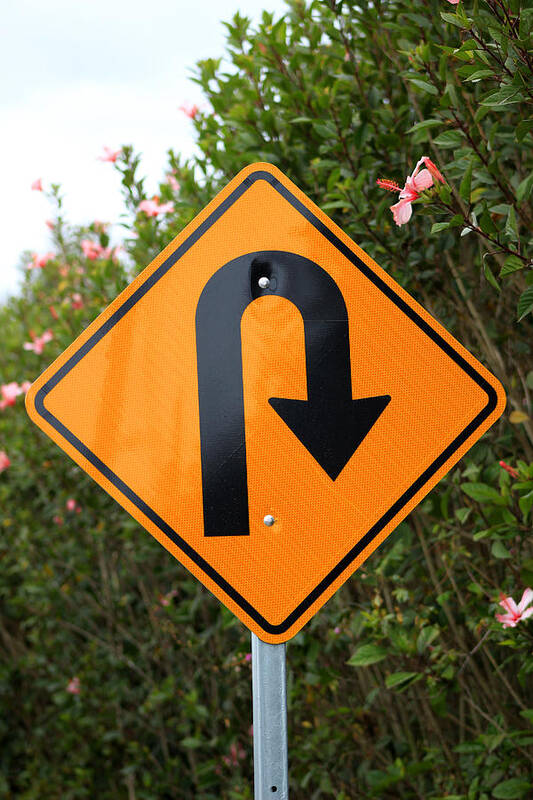The photograph depicts a vibrant outdoor scene captured during the day in natural light. Dominating the lower center of the vertically rectangular image is a silver metal pole, atop which sits a yellow diamond-shaped street sign with a black border. The sign features a black arrow indicating a U-turn that curves to the right, suggesting that this location is outside of the United States. Surrounding the pole are lush green plants and leaves, interspersed with blooming pink hibiscus flowers. The background is composed mainly of verdant foliage, while the upper left corner of the image reveals patches of blue sky and white clouds. The overall composition blends the structured form of the street sign with the organic beauty of the blooming plants and expansive sky.